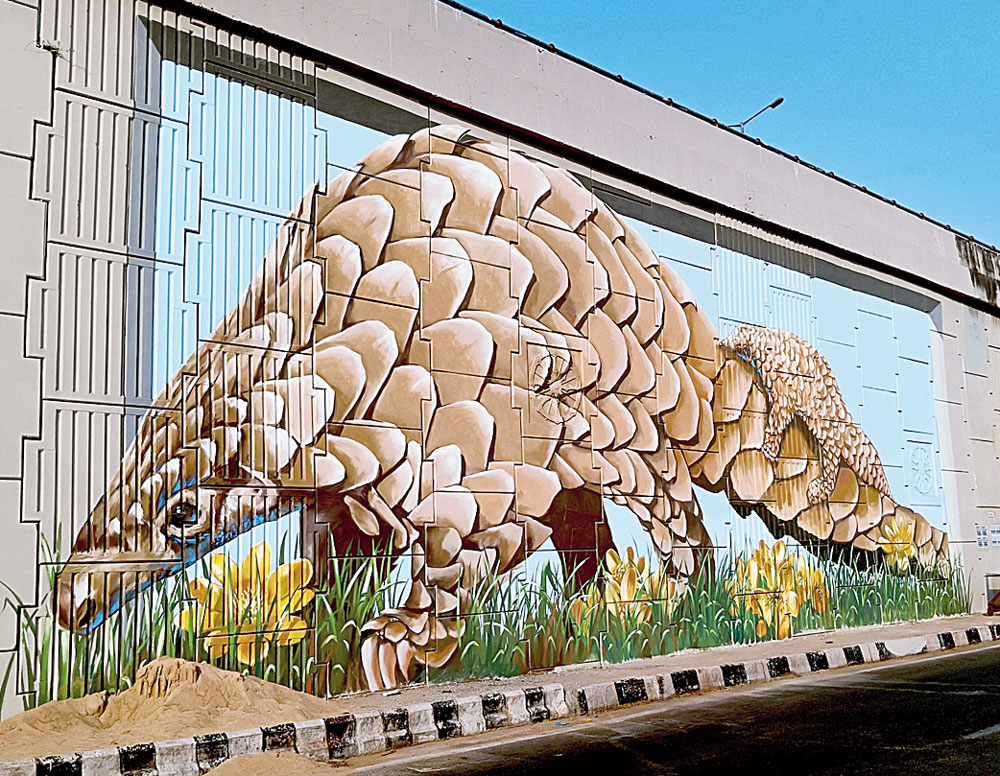The photograph showcases a large, hand-painted mural on the side of a concrete building, potentially adjacent to a roadway. The mural features a detailed depiction of a brown armadillo with an infant armadillo clinging to its tail. Both armadillos exhibit a distinct plated, armored appearance. The armadillos appear to be walking through green grass adorned with yellow flowers, which are intricately painted below them. The background of the mural is a light blue, seamlessly blending into a bright blue sky above, casting ample daylight onto the scene. The mural spans roughly 14 feet by 20 feet, taking up a significant portion of the wall. Below the mural, there appears to be a sidewalk adjacent to the painting, suggesting that people can park nearby to view this unique artwork up close. The overall scene does not feature the sun but is brightly lit, highlighting the vibrant details of the mural.